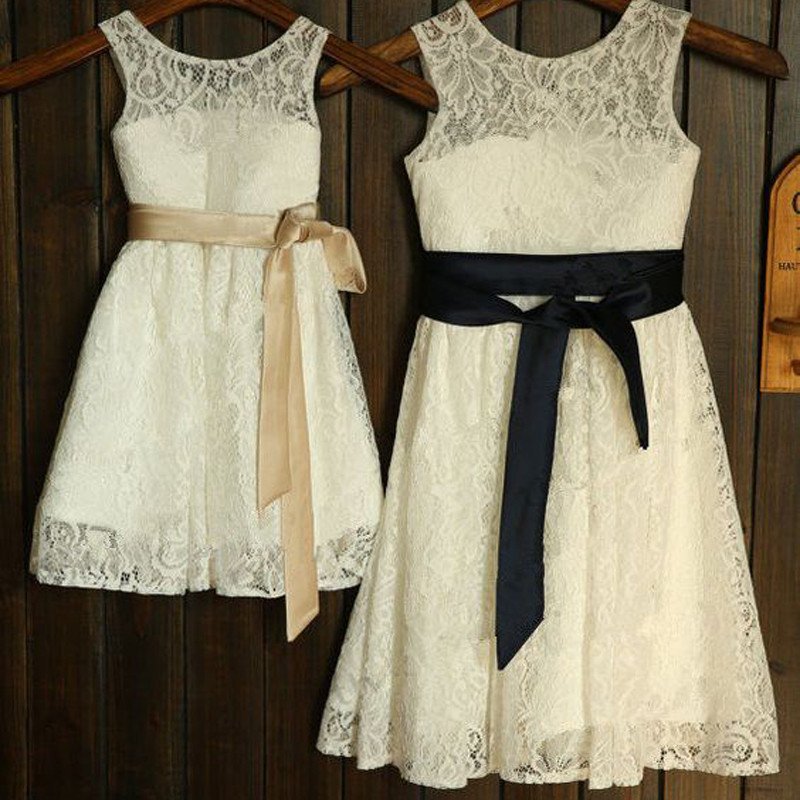In this photograph, two sleeveless, lace-like dresses are hanging side by side on matching wooden hangers against a dark wooden wall. They share an elegant design with sheer fabric around the shoulders and a floral pattern adorning the top and bottom. The dress on the right is larger, suitable for an adult, and features a loosely tied black ribbon around the waist. In contrast, the smaller dress on the left, which is about 75% the size of the larger one, likely intended for a child or a flower girl, has a fully tied gold ribbon. Both dresses are ivory or off-white in color and display a high neckline. To the right, there is a small sign attached to the wall.